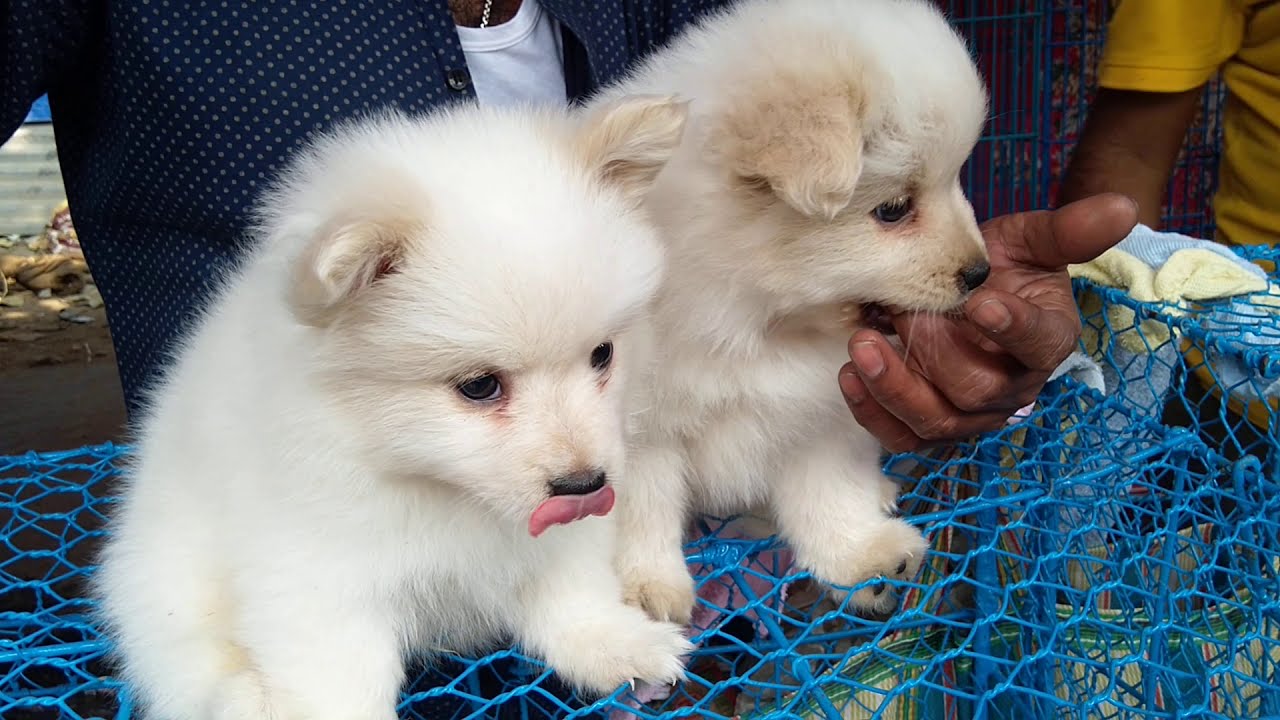The image showcases two small, fluffy white puppies, resembling Samoyeds, sitting closely together on a blue chicken wire net. The puppies, appearing to be around eight weeks old, exude an adorable and playful vibe. The puppy on the right is gently nibbling on a human hand that is cupped beneath its mouth, possibly offering food, while the one on the left has its tongue playfully sticking out. Behind the puppies, there are two people. One person, wearing a short-sleeved blue shirt with white dots over a white t-shirt and a silver chain, is more prominently visible. The other individual, standing to the right, sports a mustard-colored t-shirt and is holding a blue and yellow towel. The backdrop of blue mesh and the presence of these individuals add context and warmth to this endearing close-up scene.